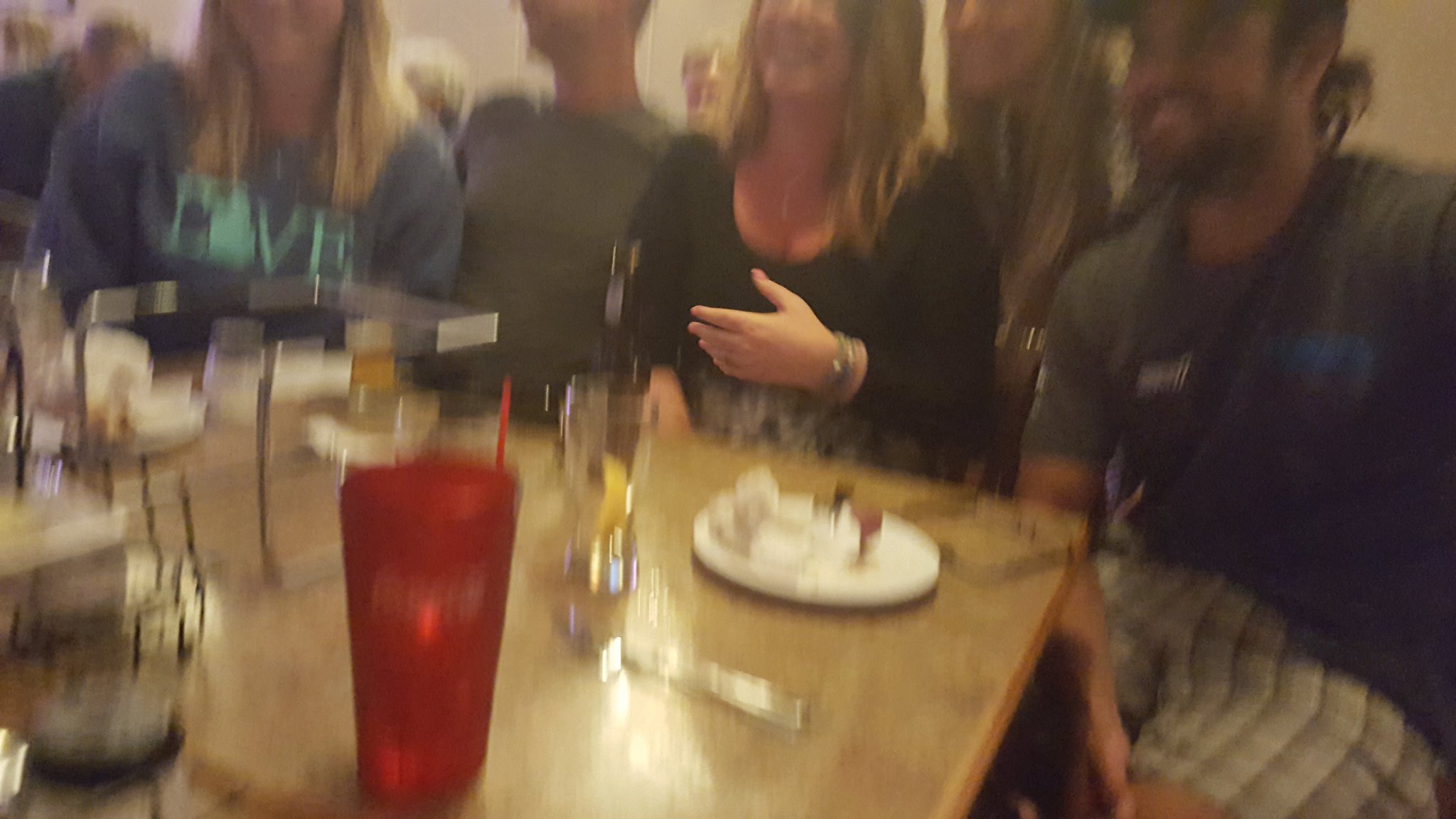This image depicts a slightly wider-than-tall, blurred, low-resolution photo of a group of five people in their 20s to 30s seated around the lower right-hand corner of a rectangular, wooden restaurant table. The scene appears to capture them mid-meal, indicated by the plates, glasses, silverware, and scattered remnants of food and drinks on the table, including a notable red Coca-Cola cup with a straw and an empty glass with a lemon slice. The composition features an Indian man on the right in an olive-green shirt, a woman next to him in a black shirt with silver bracelets, another man in a gray t-shirt, and a woman in a blue shirt with light blue lettering and long blonde hair. They all appear to be smiling and engaged, suggesting a lively, social setting. The background suggests a busy restaurant environment, enhancing the casual, spontaneous nature of the photograph.